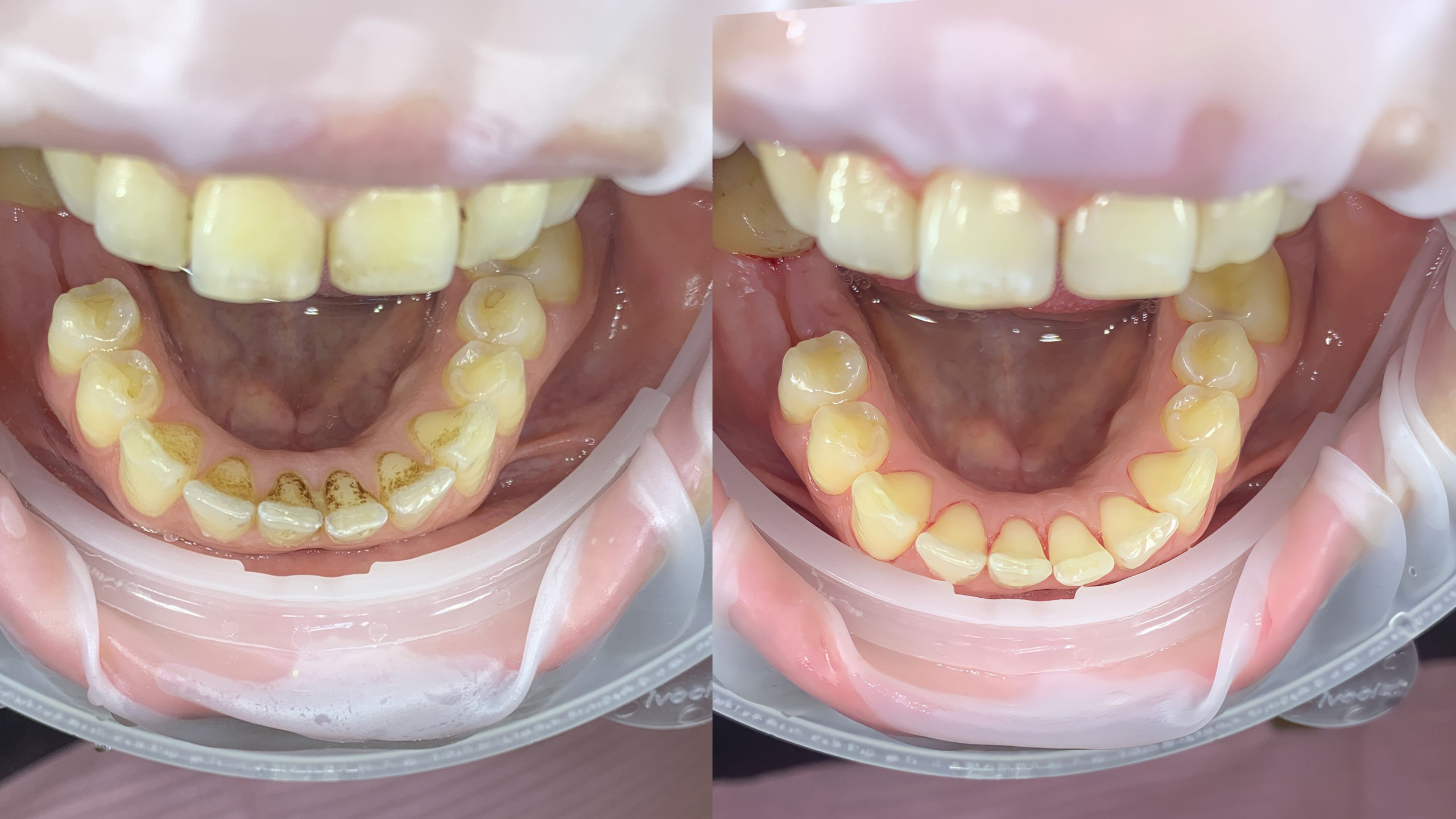In this detailed photograph, the inside of a person's mouth is shown in two side-by-side images focusing on the lower jaw and teeth. Both images are taken indoors, likely in a dental office, and feature the same pink lips, white and yellow teeth, and other intraoral structures. The person's mouth is held open by a plastic appliance, exposing the full dental view for each shot. 

On the left, the "before" image reveals teeth that are heavily discolored with significant plaque accumulation and dark cavities, particularly noticeable on three bottom middle teeth. The teeth appear dirty and exhibit obvious signs of neglect. In contrast, the "after" image on the right showcases the same set of teeth, now fully cleaned, whiter, and free of any dark spots, plaque, or tartar buildup, indicating successful dental treatment. The images are placed side by side, allowing for a clear and direct comparison that highlights the dramatic improvement in dental hygiene.